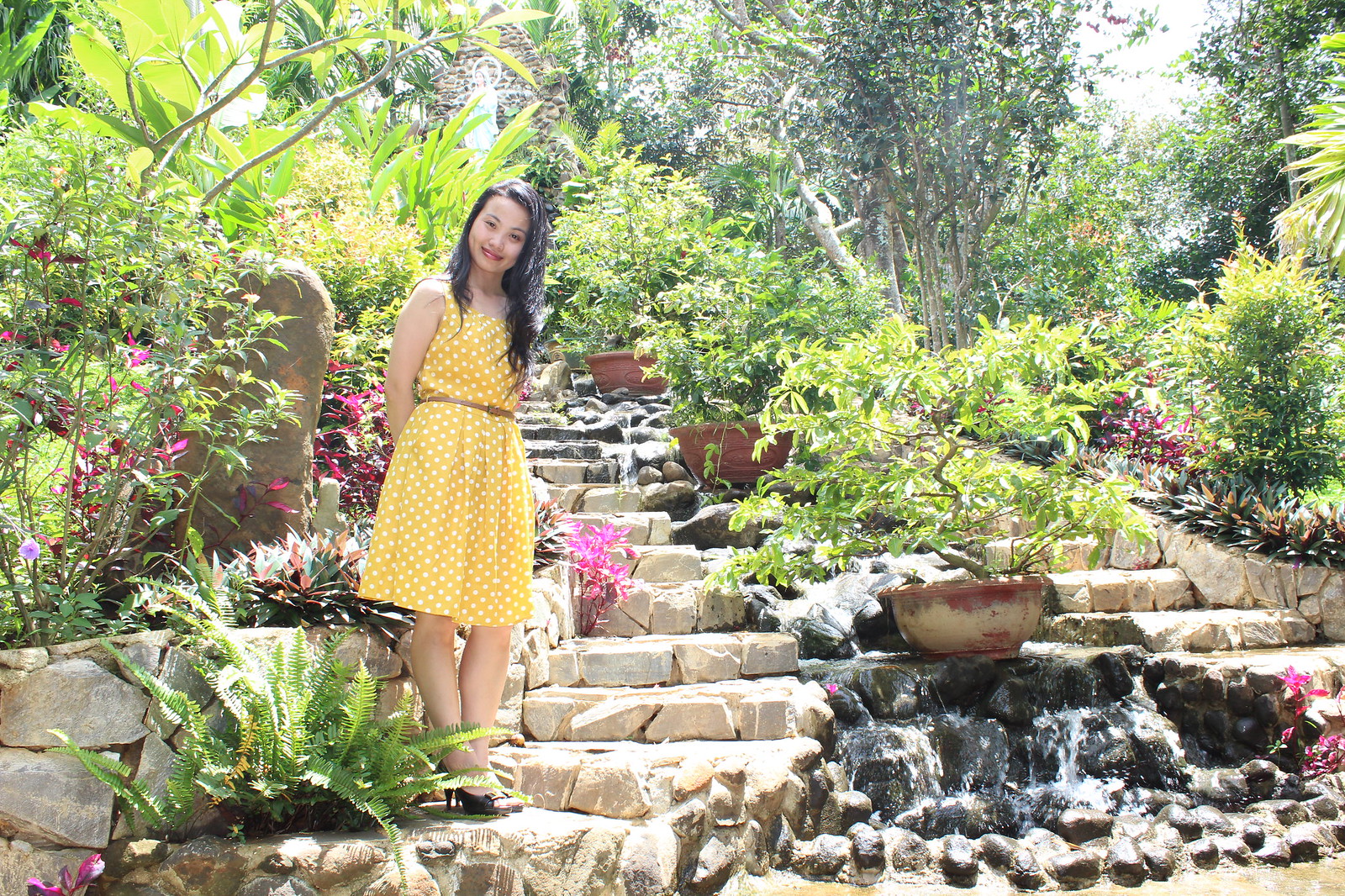A woman stands gracefully on rocky steps amidst a stunning hillside garden display. The steps, crafted from small boulders, flank a charming garden pot that sits centrally, containing a lush, bonsai-like plant with vibrant green leaves. A gentle stream of water cascades down the middle of the stairway, adding a serene element to the scene. The area is adorned with a rich variety of trees and foliage, complemented by scattered clay pots that contribute to the picturesque waterfall landscape. The woman, dressed in a light yellow dress with white polka dots and high heels, smiles warmly at the camera, her long hair cascading around her. She tilts her head slightly, exuding a sense of joy and tranquility. Her appearance suggests she may be of Asian descent, enriching the cultural aesthetic of the image.